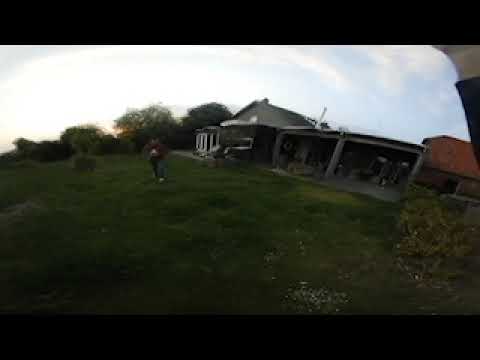This image depicts an outdoor scene that appears to be the yard of a home, characterized by a lush, green landscape with grass, trees, and bushes. The visual quality is noticeably poor, with the image appearing heavily compressed and out of focus. Centered in the yard is an indistinct figure, likely wearing blue jeans and a burgundy hoodie, engaged in an unclear activity. The house itself is a gray structure with two garages on the right side, featuring a distinctive porch with white columns on the left. Adjacent to the garages is a red-roof barn or shed. The yard also contains some landscaping elements, including a bush in the lower right corner and a few white specks scattered around. The image is framed by horizontal black bars at the top and bottom, adding a widescreen effect, and captured under daylight conditions, suggesting it was taken from someone's front lawn. The overall atmosphere of the yard is somewhat unkempt yet vibrant with greenery.